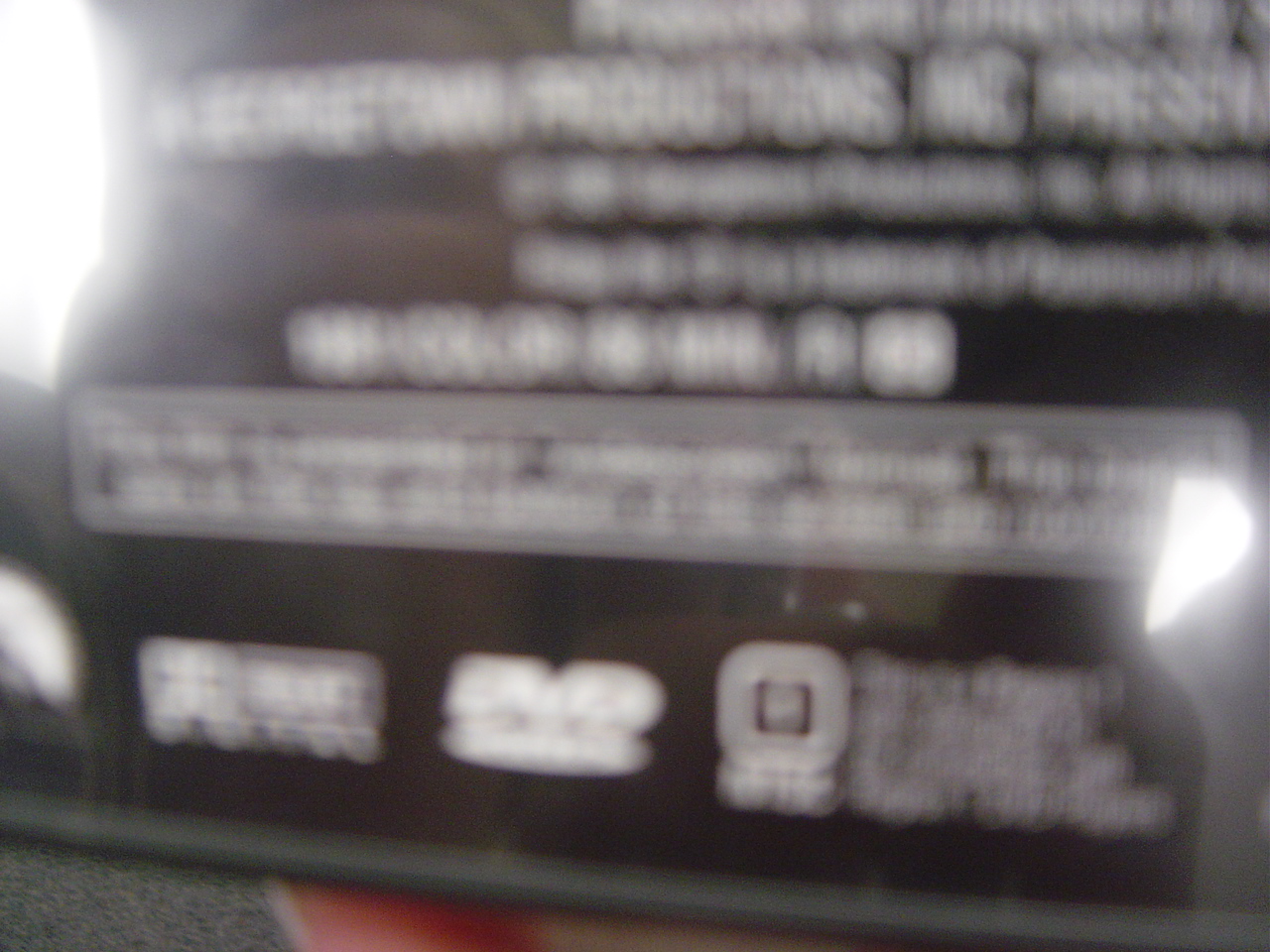This image depicts a very blurry photograph of what appears to be the back of a DVD package. The picture is severely out of focus, rendering the printed text largely illegible. At the bottom center of the image, the word "DVD" is faintly discernible. The package has a shiny surface, evidenced by two bright spots of reflected light—one on the right side and another in the top left corner. The dark background features multiple lines of white text, including a prominent rectangular box of text situated in the middle of the image. Despite the blurriness, the overall layout suggests typical informational content found on DVD packaging.